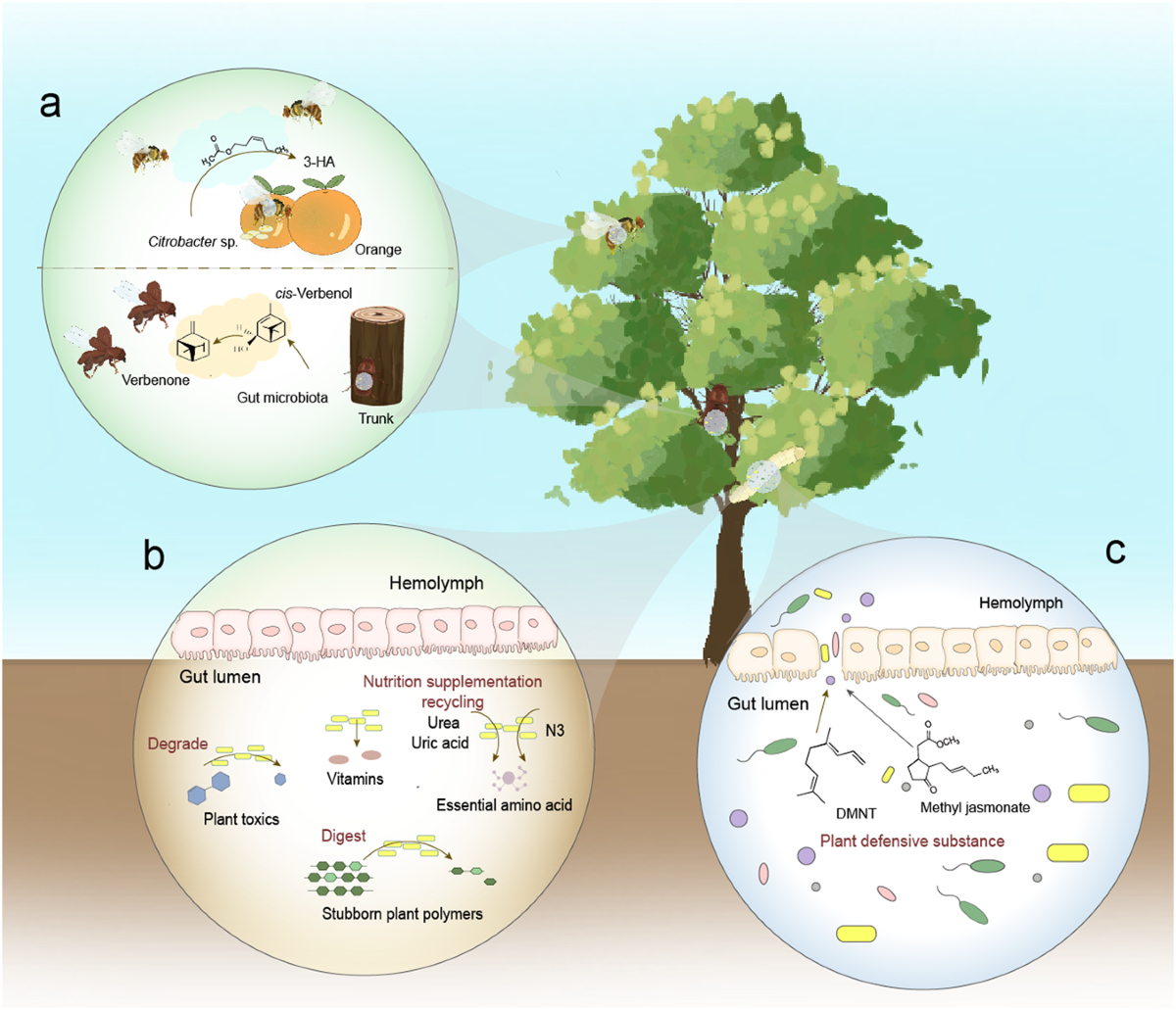The image is a digitally illustrated diagram of a tree, depicted within a light blue sky and light tan ground. This central hardwood tree, with clusters of dark green, greenish-gray, and yellowish-green leaves, is positioned just to the right of center in a square frame. Surrounding the tree are three large circles labeled A, B, and C.

Circle A, located just to the left of the tree, contains various elements including a picture of an orange at the top and the label "Citrobacter sp. 3HA." It also features the terms "CIS Verbinol," "Gut Microbiota," "Trunk with Verbinone," and illustrations of foods reacting within the context of human nutrition. There is a depiction of a brown flying insect positioned by the tree trunk.

Circle B, positioned centrally, is packed with intricate details like molecular or cell diagrams. It labels terms such as "Hemolymph," "Gut Lumen," "Nutrition Supplementation Recycling," and "Plant Toxics." Additional key words include "Urea," "Uric Acid," "N3," "Vitamins," "Essential Amino Acids," "Stubborn Plant Polymers," and "Degrade," providing a comprehensive depiction of nutritional and digestive processes.

Circle C, on the right, similarly features molecular diagrams and is labeled with "Hemolymph," "Gut Lumen," "DMNT," and "Methyl Jasminate." At the bottom, it prominently displays the warning "Plant Defensive Substance" in red, underscoring the defensive chemicals associated with the tree.

The diagram intricately ties together the ecological and biological interactions involving the tree, various microorganisms, and defensive substances, offering a detailed and visually rich representation.